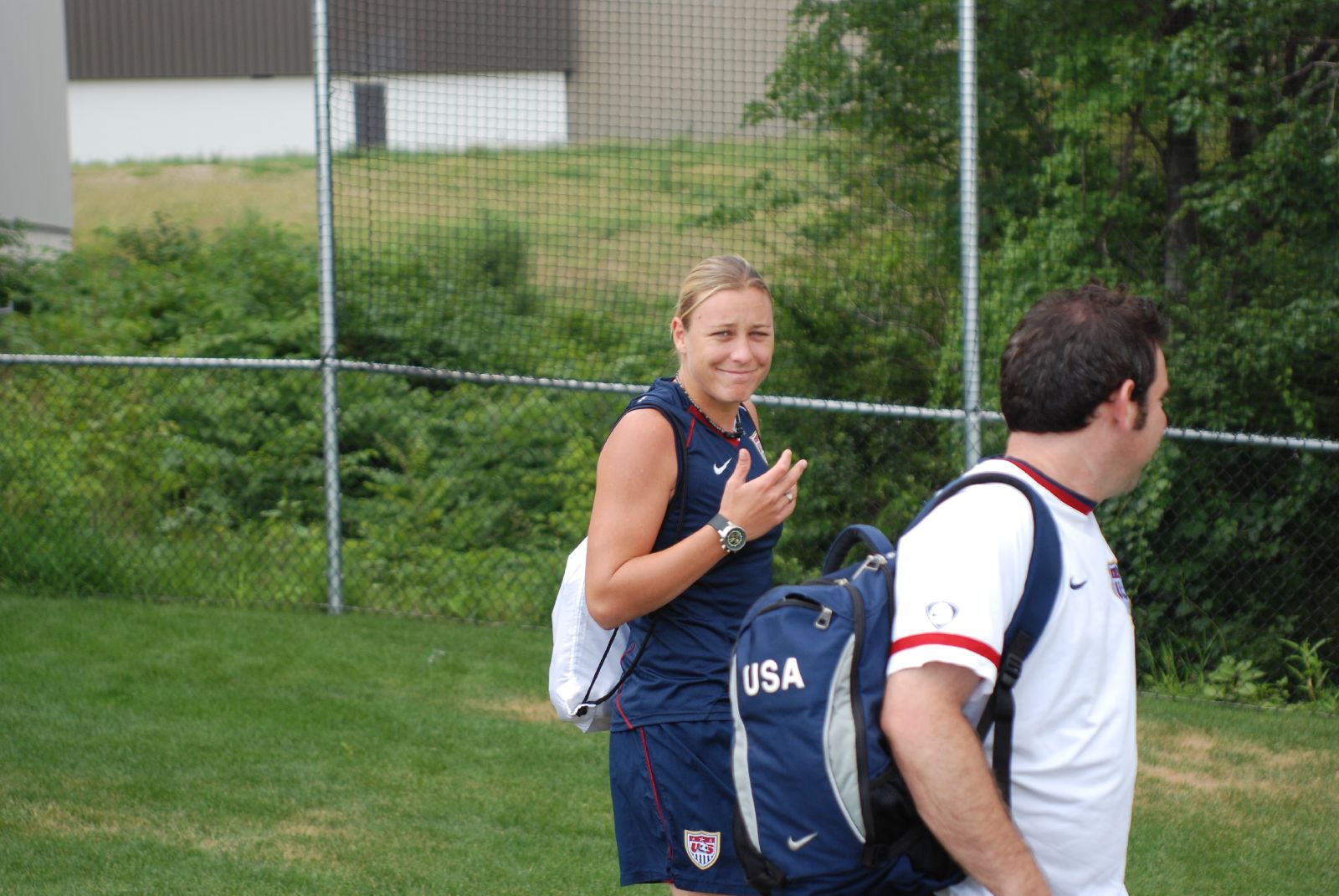In this detailed outdoor photograph taken on a grassy field, we see a female athlete and a male companion walking together. The young woman, a white female with blonde hair, is central to the image, smiling directly at the camera. She sports a blue athletic uniform, consisting of a sleeveless tank top featuring a white Nike logo on the right chest, and matching blue shorts with a red stripe down the side. She carries a white nylon backpack on her back and wears a watch on her right wrist. Next to her, but partially turned away, is a white male with black hair. He is dressed in a white t-shirt that also has a blue Nike check mark, accented with a red collar and red stripes around the sleeves. His blue backpack, emblazoned with "USA" in white letters, is slung over one shoulder. The scene is set in broad daylight, with the duo walking along a flat, grassy area bordered by a tall chain-link fence. Beyond the fence are trees, green bushes, and additional grassy patches, and a black and white building can be seen in the distant background. The image conveys a sense of casual athleticism, capturing the two figures in mid-stride amidst a serene, outdoor setting.